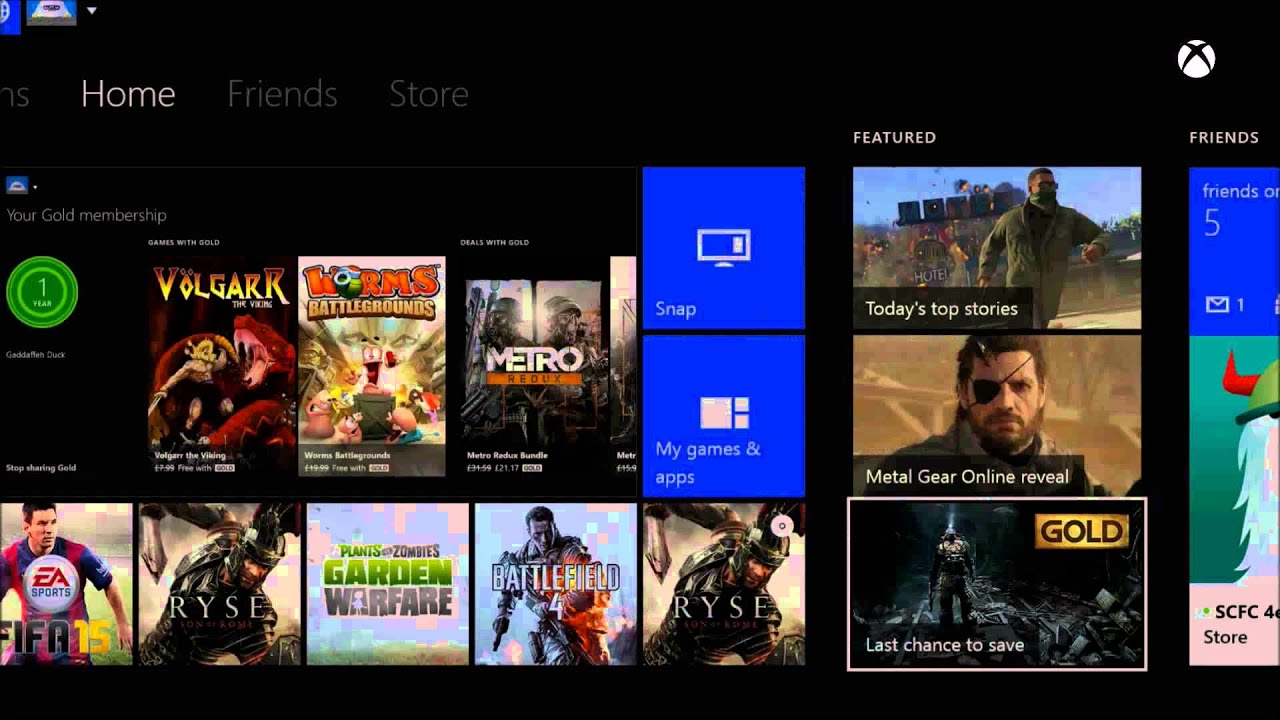This screenshot captures the interface of an Xbox home page, teeming with various movie snippets and application sections. The interface prominently showcases the "Home" tab, which is highlighted in white at the far right. This tab confirms the user is on the home page where a plethora of movies and exciting features are showcased, including up-and-coming releases. 

A distinguishable Xbox logo graces the top-right corner, reinforcing the platform’s identity. Below "Home," the user's gaming status is displayed, confirming their "Gold Membership." The username floats above this section, with a "One Year" subscription period indicated in green, suggesting an annual membership.

Directly underneath this membership information, several movie titles are listed. Notably, there is a movie titled "Vulgar," priced at $7.99; however, this price is crossed out, indicating it’s free for Gold members. Additionally, blockbuster games such as "Worms Battlegrounds" and "Metro Redux" are featured. Beneath these are more game titles, starting from the left: "FIFA 15," "Ryse: Son of Rome," "Plants vs. Zombies," "Battlefield 4," and another "Ryse: Son of Rome."

At the top, two prominent blue boxes are visible. One contains a snap feature with a TV icon, while the other is for "My Games & Apps." 

To the right of these boxes is a column dedicated to "Today's Top Stories," showcasing important updates like the "Grand Theft Auto" image and the "Metal Gear Online reveal." Currently, the "Last Chance to Save" is highlighted in this section.

Lastly, the "Friends" tab is situated to the far right, featuring a dedicated box that directs users to view their friend's activities and interactions.